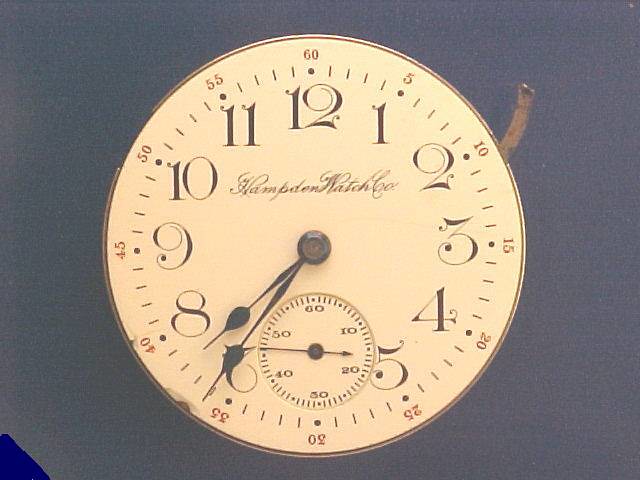This image depicts an ornate clock from the Hampton Watch Company. The clock face features elegant numerals from one to twelve, with each number crafted in intricate script. Uniquely, at the six o'clock position, there is a secondary, smaller clock, possibly designed to track seconds. Surrounding the main numerals, additional red numbers increment in fives, such as 5, 10, 15, and so forth. The clock's hands exhibit an elaborate design: they start as thin lines, expand into a teardrop shape, and then continue as a narrow line. "Hampton Watch Company" is inscribed in a flowing script across the tan backdrop of the clock, the text written in a rich brown hue. Metallic components protrude from the clock's rear, extending straight up. A noticeable chip mars the bottom left corner of the clock's face, where there's also a hint of something blue visible in the background.